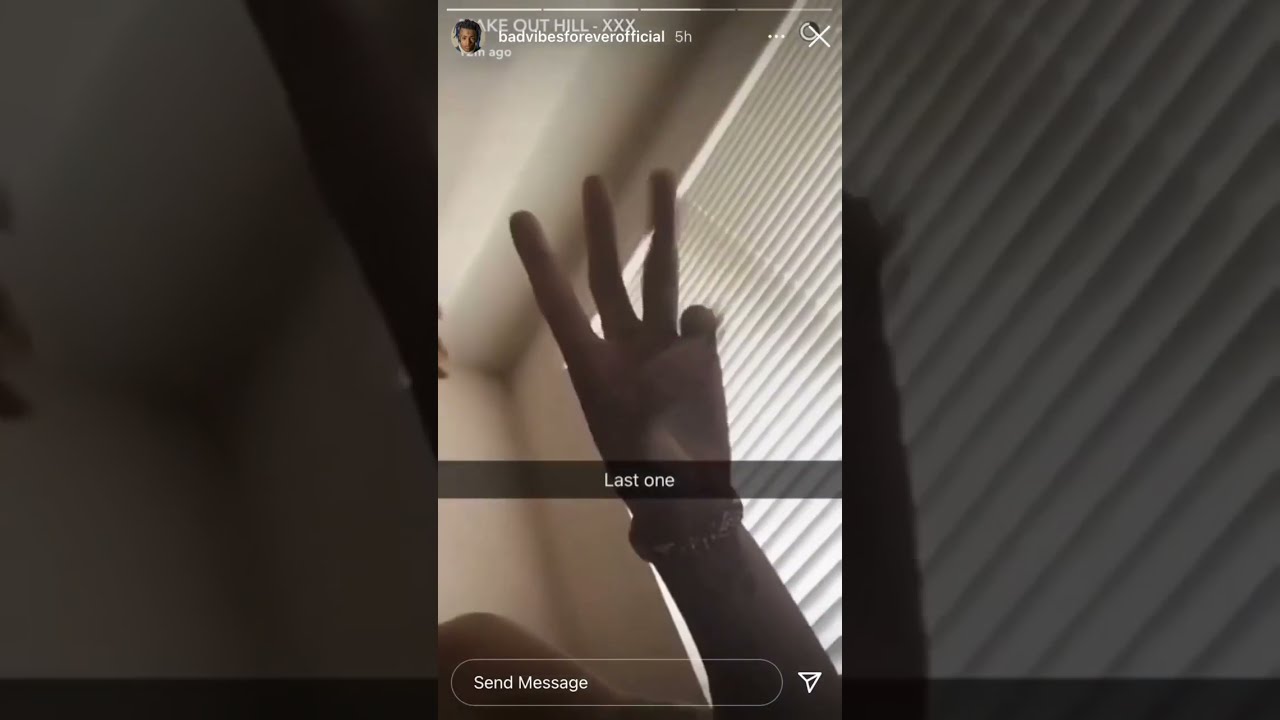This photograph captures an Instagram story mid-view, indicated by the presence of thin, white progress bars at the top. Halfway through the third segment, the story header reads “Makeouthill-XXX” followed by an icon of a person and the text "Bad Vibes Forever Official 5 hours". In the upper right corner, there's an X button for closing the story. The central focus of the image is a hand with the index, middle, and ring fingers extended, while the thumb and pinky are folded in. Behind the hand, we see part of a window with white blinds, a ceiling, and a back wall, suggesting the photo was taken indoors. Over the hand, a semi-transparent dark gray rectangle displays the caption “Last One” in white font. At the bottom of the photo is a rounded, stadium-shaped button with a paper airplane icon, labeled "Send Message." The left and right borders of the image are overlaid with enlarged and faded elements of the main picture, adding a stylistic frame to the story.